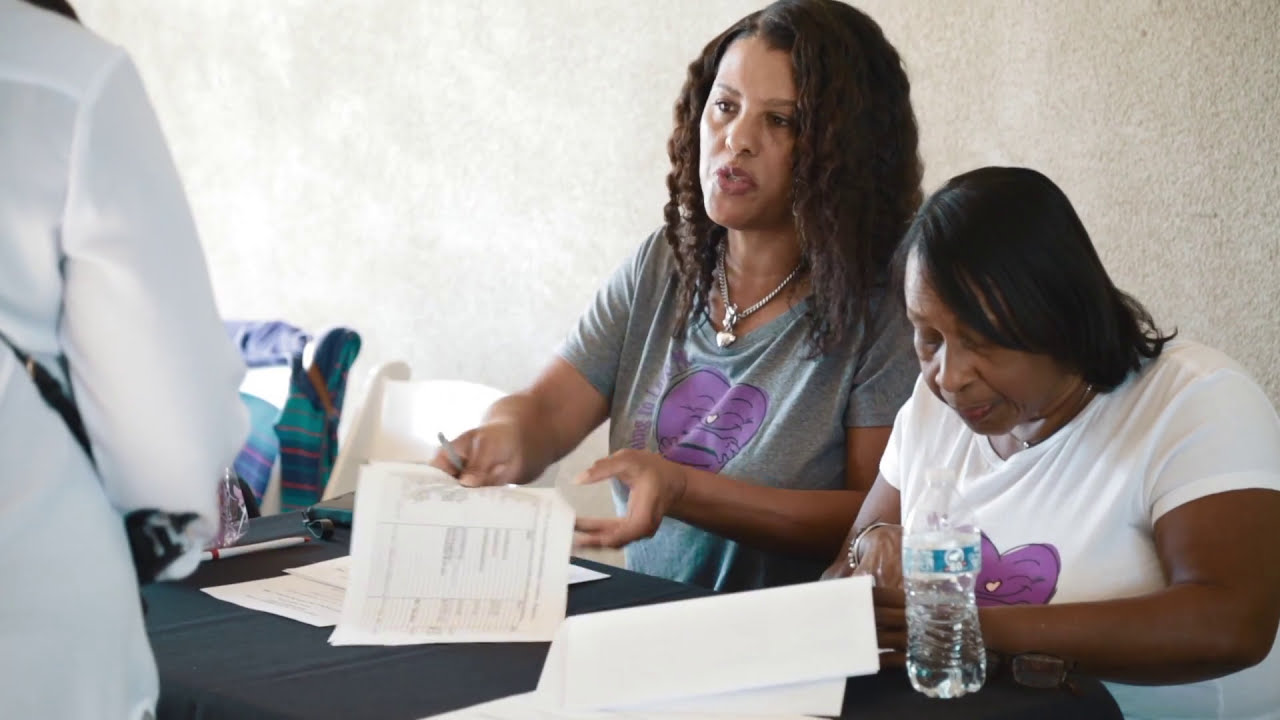The photo captures a scene at a check-in table where two African-American women are seated, engaging with paperwork. The table, covered with a black tablecloth, is positioned towards the bottom left of the image. To the far left, partially visible, is a person standing, wearing a white shirt or jacket, with a black belt, turned away from the camera.

The woman on the left has wavy, shoulder-length brown hair, and is wearing a gray t-shirt with a purple logo depicting a heart figure. She also wears a silver necklace and is in the process of handing a sheet of paper, possibly filled with contact information, across the table. She holds a pen in her right hand, and her mouth is slightly open, suggesting she is speaking.

The woman on the right, who has smooth, straight black hair and darker skin, is wearing a white t-shirt with the same purple logo. She is also adorned with a necklace and is focused on the document in front of her, consulting it intently. A water bottle sits on the table to her left, positioned near some scattered white sheets of paper. Both women appear to be engaged in an administrative task, possibly a check-in process or registration.